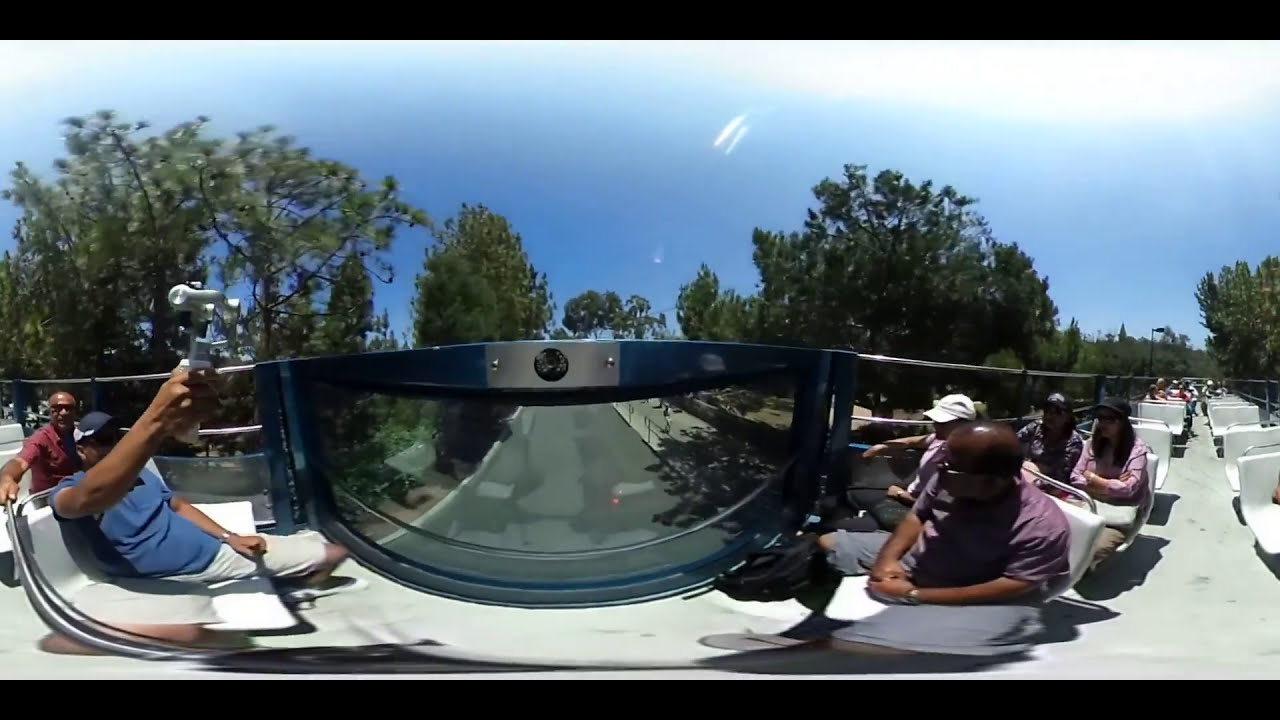A daylight image showcases a bustling, open-top tour bus filled with passengers enjoying a scenic ride. The bus features white, bench-style seating with sleek, silver frames and glass panes along the sides. At the front of the bus, a man wearing a blue shirt, cap, and white shorts is holding a silver, circular device in his right hand, likely a camera. Directly behind him, a bald man in a maroon shirt and gray shorts is wearing black sunglasses with a silver frame. 

On the right side, another bald man, sporting a purple shirt and glasses, sits next to a person in a light-colored shirt and dark pants. Further back, two women in pink or purple shirts with black hats and sunglasses are seated. The bus is driving down a dark, gray and light gray street lined with trees, green foliage, and a white curb on either side.

In the wider scene, the sky is a gradient from white to light blue, with trees lining the street on both sides. The crowded bus and the backdrop of green trees and clear blue sky create a lively and vivid touristic atmosphere.